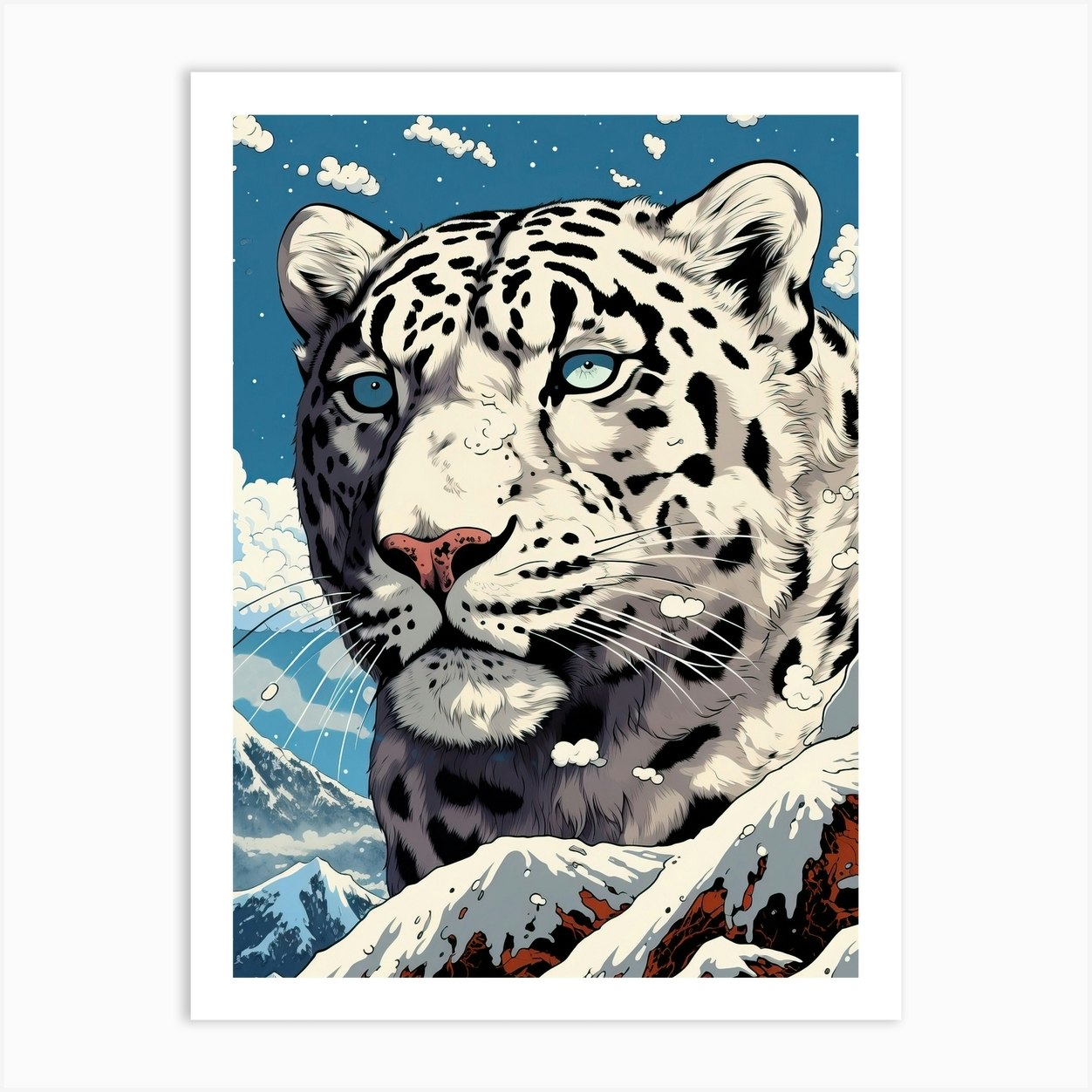This vibrant poster presents a multi-layered artistic portrayal of a snow leopard. The overall image is vertically rectangular, framed by a white border on a grey background. Dominating the composition is the head of a white leopard, distinguished by its black spots and an engaging expression. The leopard's ears are perked up, and it features a striking mix of one green eye and one blue eye, the latter subtly darker, possibly due to shadows. Its red nose and delicate whiskers add a touch of realism to the face.

In the background, the sky is a deep blue adorned with soft white clouds and faint stars, which enhances the celestial atmosphere. Snow-capped mountains in shades of gray and brown stretch across the lower part of the image, their peaks covered in snow, contributing to a cold, wintry ambiance. Smaller clouds drift in front of the leopard's face, further enriching the scene. This detailed drawing masterfully blends the majestic presence of the snow leopard with the serene, frosty landscape, creating a striking visual narrative.